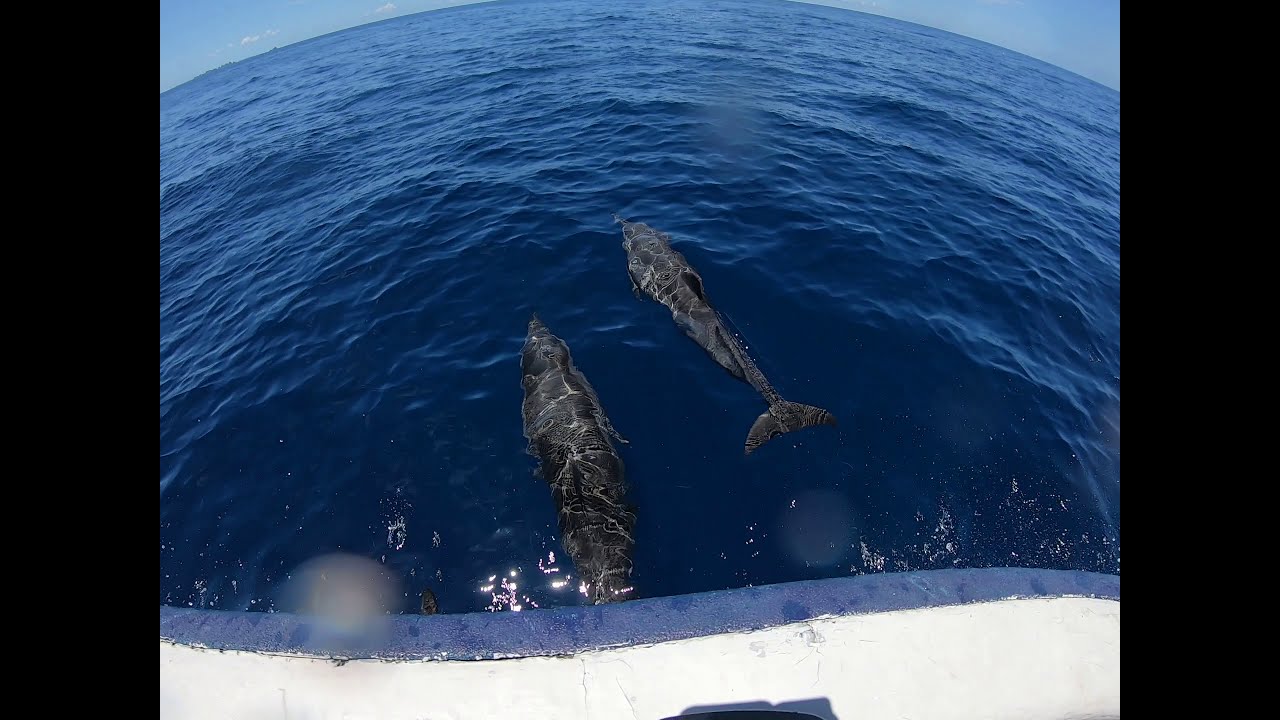Taken from a boat, the photograph captures a vast, clear ocean with a concave appearance due to the viewer's perspective. The bottom of the image features white structures indicative of the boat. Blurry spots, likely water droplets on the camera lens, are also present. In the center foreground, two dolphins swim gracefully close to the boat, unafraid and familiar with human presence. One dolphin appears smaller, suggesting a mother and calf duo. The expansive, blue ocean and visible waves form the backdrop, along with a partially cloudy sky adding depth to the scene. The prevalent colors are blue, white, and shades of gray, emphasizing the serene maritime setting.